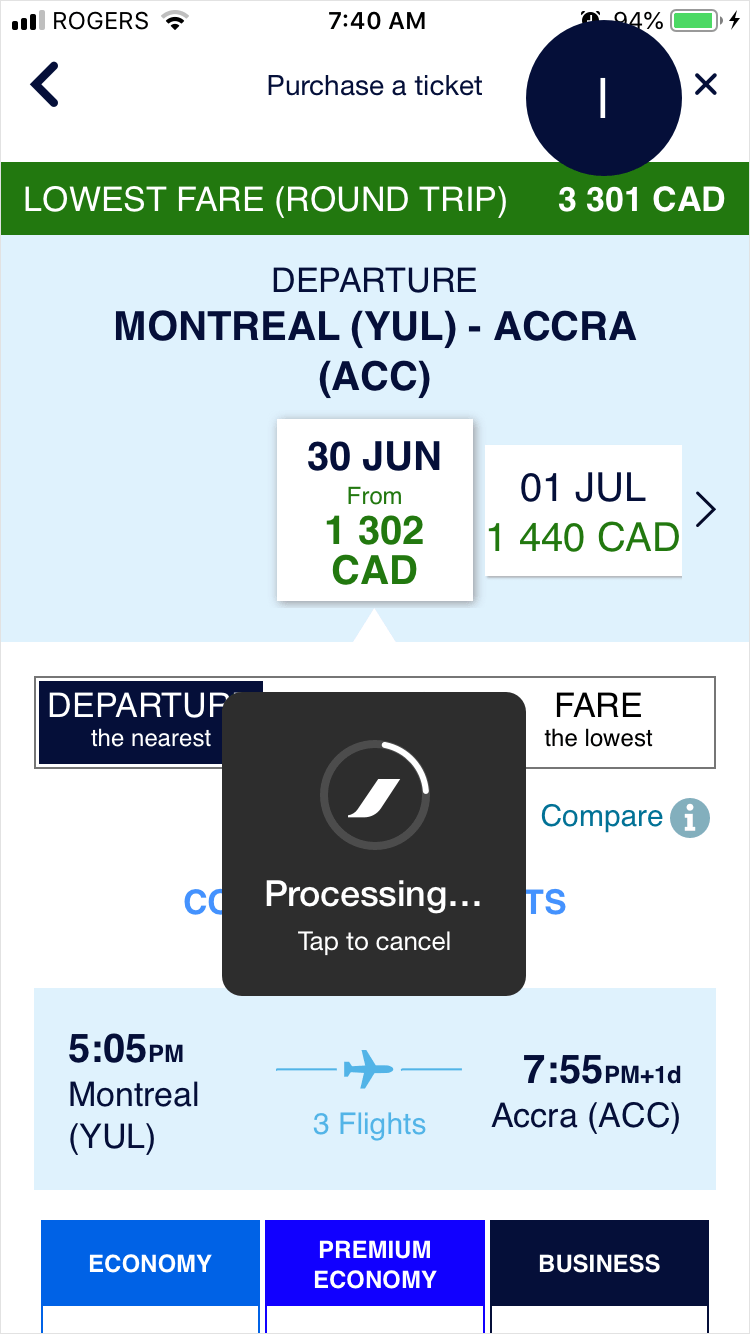The screenshot displayed is from a mobile flight booking application. At the very top of the screen, the user is on the "Purchase a Ticket" page. Beneath this header, there's a labeled section indicating "Lowest Fare Round Trip," priced at 3,301 CAD (Canadian dollars). The flight being booked departs from Montreal and arrives in Accra (spelled A-C-C-R-A), with the selected departure date being June 30th. 

During the booking process, a prominent message reading "Tap to Cancel" suggests that the transaction is currently processing. Further down, the screen details the flight itinerary, stating a departure time of 5:05 PM from Montreal. The journey includes three connecting flights, culminating in an arrival at Accra at 7:55 PM the following day. At the bottom of the screenshot, options for different seating classes—Economy, Premium Economy, and Business—are visible, although it is unclear which class is selected due to cutoff information.